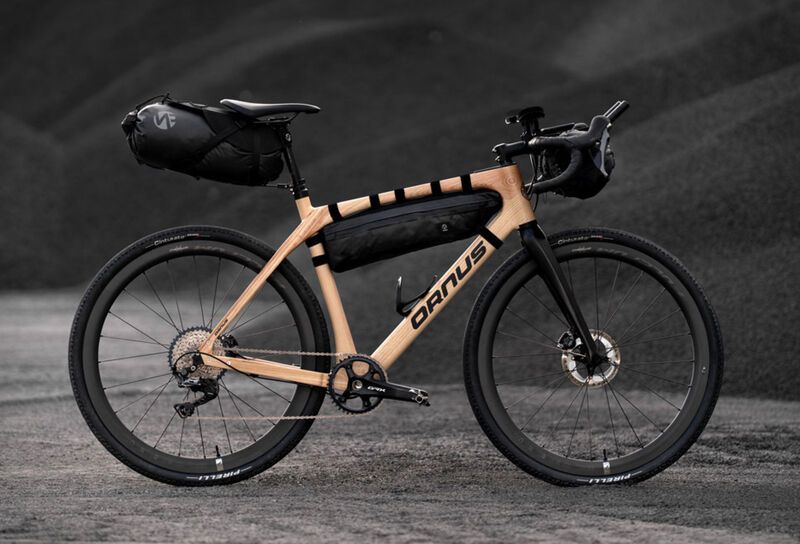This image depicts a side view of a bicycle set against a dark gray, hilly backdrop. The bicycle is notable for its large black tires, which feature intricate, thin gray wire patterns. A silver gear connects to a frame in the lightest imaginable shade of orange, with a subtle brown tint. At the center of the frame is a black gear, and the frame prominently displays the company's name, ORNUS. Positioned beneath the gray seat is a mini black duffel bag, adding a touch of practicality to the bike's design. The front section of the bicycle is black, seamlessly blending into the overall color scheme. The bicycle rests on a bed of gray gravel, completing the detailed setting of the scene.